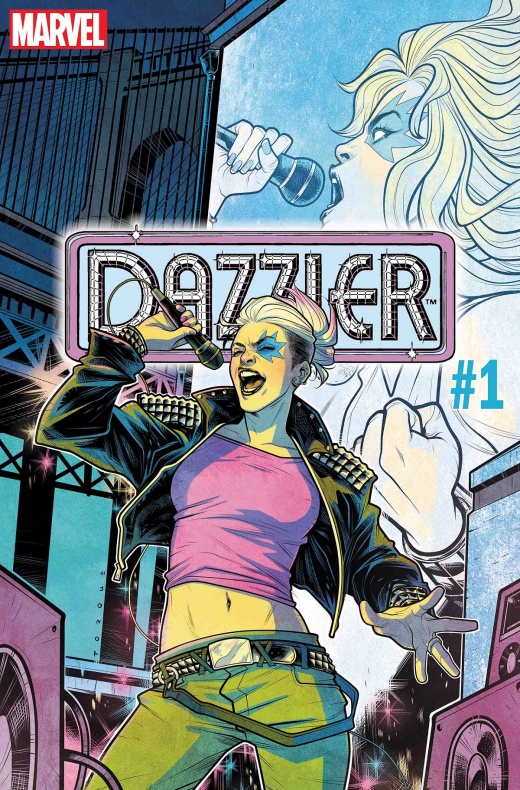The cover of this Marvel comic book, titled "Dazzler Edition 1," prominently features a dynamic scene with a central animated woman deeply immersed in her performance. The classic red and white Marvel logo is situated in the top left corner. The title "Dazzler," written in glimmering, diamond-like text framed by a pink border resembling a license plate, draws attention in the middle of the cover. The central figure, presumably Dazzler, exudes a rockstar aura with her white hair highlighted with pink streaks, a star painted on her right eye akin to David Bowie's iconic look, and her intense expression with closed eyes as she belts out a song into a microphone. She dons a studded black leather jacket over a pink crop top, paired with either jeans or black pants, and a studded black belt with a metal buckle. Surrounding her on the stage are pink speakers, enhancing the concert vibe. Overlaying the scene, at the top right, is an image on what appears to be a billboard or marquee showing another woman—also adorned with similar star eye paint but with blonde hair—singing, capturing the essence of an ongoing performance and highlighting Dazzler as a mesmerizing musical artist.